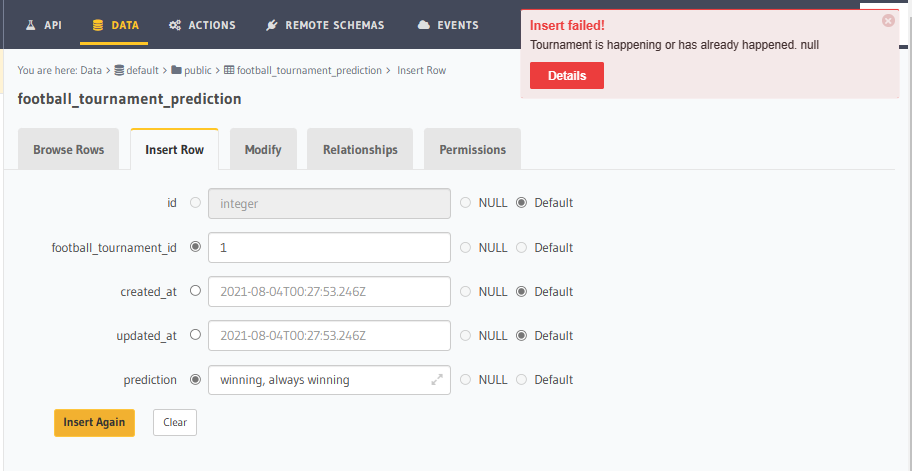Here is a detailed and clean caption for the image described:

---

The screenshot showcases an API interface against a black background, with the word "Data" highlighted in orange and underlined. The interface transitions to a white background featuring several hierarchical navigation elements indicating the user's current position: "You are here: Data > Default > Public > Football > Tournament > Prediction > Insert Row."

In bold, black text, underlined titles "Football," "Tournament," and "Prediction" are presented above a series of interactive options. Users can browse rows using a gray box or insert a row through a white box with an orange header labeled "Insert Row." Adjacent to it, gray boxes labeled "Modify," "Relationships," and "Permissions" offer additional functionalities.

The form fields include:
- **ID Integer** (default value)
- **Football Tournament ID** (value set to 1)
- **Updated At** (default value)
- **Prediction** (text input: "winning, always winning")

At the bottom of the form, users can choose to finalize the insertion with an orange "Insert" button or clear the form using a white "Clear" button.

At the top right corner of the interface, an error message reads, "Insert failed: Tournament is happening or has already happened," accompanied by a red "Details" button.

---

This caption provides a clear, detailed description of the interface and its elements.